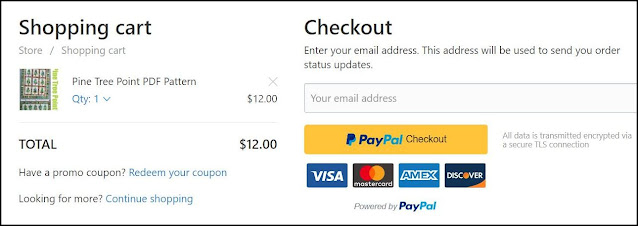A detailed view of an online shopping cart and checkout interface on a white background. The screen prominently displays a shopping cart icon alongside checkout options. The cart lists a single item with the description "Quantity: 1" in blue, priced at $12. The total cost is also marked as $12. Below the summary, there is a prompt for users to enter a promo code, with a blue link labeled "Redeem your coupon."

Additionally, there is a section encouraging users to continue shopping, highlighted by the blue text "Looking for more? Continue Shopping." Further down, there's an input field titled "Enter your email address,” specified for sending order status updates, with an example email address inside a box.

For payment, there is a "PayPal Checkout" button, and a note confirming that all data is transmitted securely via TLS encryption. Payment options include icons for Visa, MasterCard, American Express (Amex), and Discover. At the very bottom, the interface reads "Powered by PayPal."